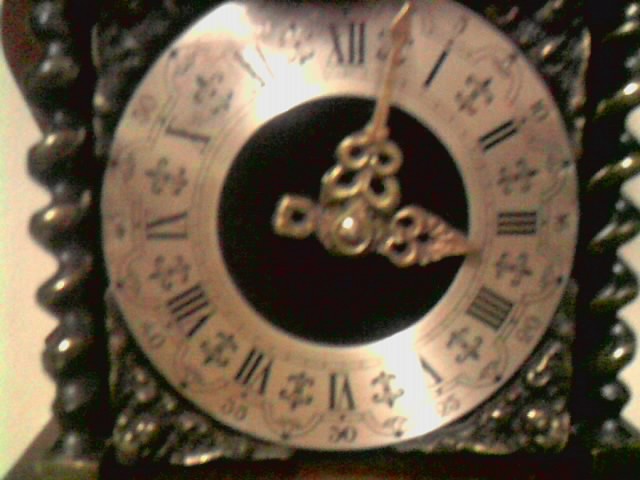This image captures an intricately designed clock with a charming vintage aesthetic. The clock appears to be framed in a structure resembling brown wood, possibly real or perhaps an artistic representation. The sides of the clock are spindly, displaying a mix of brown wood and gold accents. The backdrop of the clock is a rich, dark brown that enhances its wooden texture.

At the center of this timepiece is a prominent gold circle serving as the clock face, adorned with Roman numerals from I to XII, likely in dark brown or black. Between the numerals, there are small emblems resembling swords, adding to the clock's ornate design. The border is highly decorative, featuring intricate patterns. Completing this elegant piece are the fancy gold hour and second hands, which stand out strikingly in the middle.